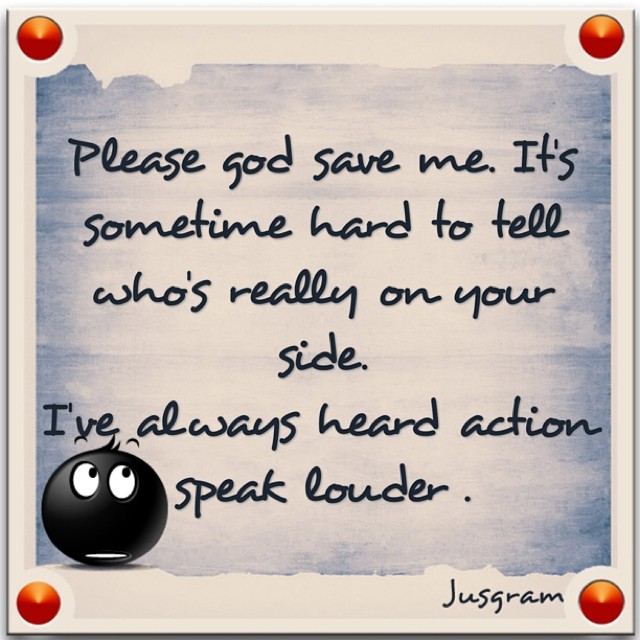This image appears to be a graphic or an ad, designed to look similar to a post-it note. The central element is a white card with a bluish-gray background where the text is written in a black, cursive, handwriting style. It reads: "Please God, save me. It's sometimes hard to tell who's really on your side. I've always heard actions speak louder." There is an artist's inscription at the bottom which reads "Jug Graham." Additionally, the image features a black, cartoonish face in the bottom left corner of the card. The face resembles a bowling ball or a bomb, with white eyes looking upward, a thin white mouth, short hair sticking up, and eyebrows positioned outside the sphere, giving it a dejected expression. Orange pushpin-like dots mark each of the four corners of the square card, adding to the post-it note aesthetic. There is no date or other identifying information present in the image.